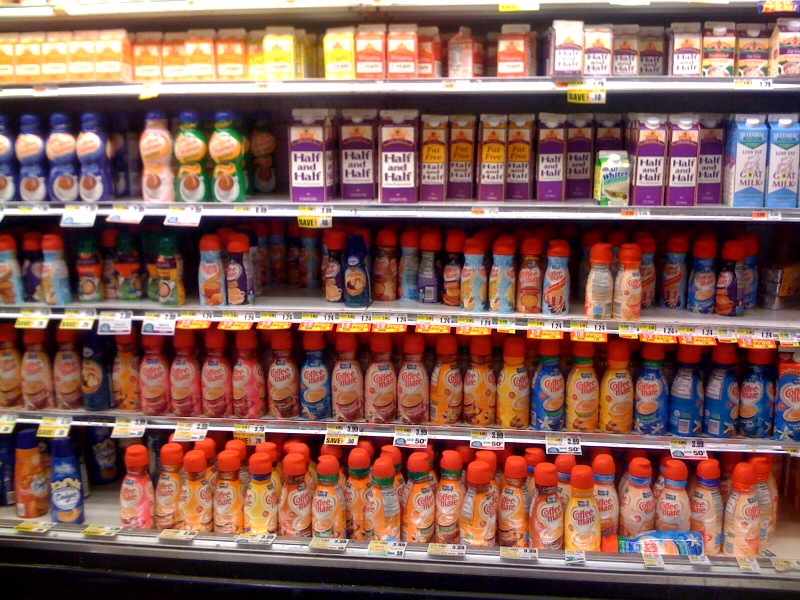The image captures a well-organized refrigerated coffee creamer section in a supermarket. There are five shelves in total, stretching across the entire frame, each brimming with an assortment of coffee creamers. The arrangement showcases a variety of sizes and colors, prominently featuring brands like Coffee Mate with bottles of various flavors in orange, blue, and yellow. The bottles are mostly capped with wide red screw tops, though some are missing, revealing occasional gaps on the shelves. The bottom three shelves are densely packed with a multitude of Coffee Mate bottles, while the higher shelves transition to cartons, primarily containing Half and Half, and some Goat Milk products on the right side. The top shelf is lined exclusively with cartons labeled as Half and Half. One notable detail is a fallen blue-labeled bottle with a red cap on the lowest shelf. The shelves appear partially organized by product type and color, with the second to top shelf showing a lesser density, possibly indicating their convenient arm-height position. Overall, this snapshot provides a comprehensive view of a supermarket's coffee creamer and milk alternatives section, replete with detailed price tags and a meticulous alignment by brand and flavor.